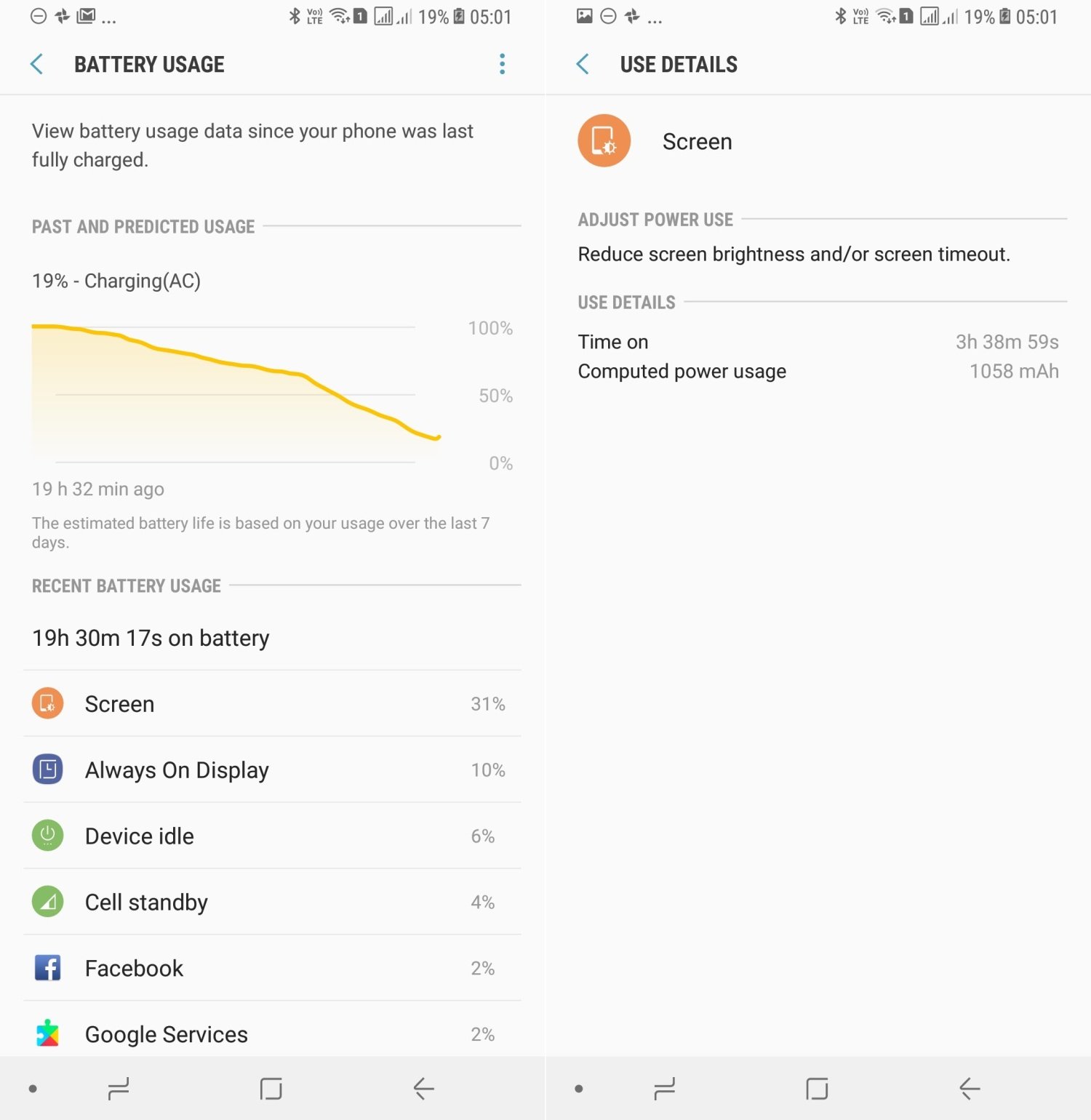The image displays two screenshots of a smartphone's battery usage details, captured side-by-side. At the top of both screens, typical smartphone status indicators are visible, including the Bluetooth status, Wi-Fi strength, network status, battery meter, and current time.

In the left screenshot, the title "Battery usage" is prominently displayed, followed by a note stating, "View battery usage data since your phone was last fully charged." It then indicates both past and predicted usage times, with the phone currently at 19% battery after being on for 19 hours and 32 minutes since the last full charge. The estimated battery life is based on usage patterns over the last seven days. Below this overview, there is a "Recent battery usage" section showing the phone has been on battery for 19 hours, 30 minutes, and 17 seconds. The breakdown of battery consumption is listed as follows: screen (31%), always-on display (10%), device idle (6%), cell standby (4%), Facebook (2%), and Google (2%).

The screenshot on the right focuses on the "Use details" of the screen's battery consumption. It advises users to "Adjust power use" by reducing screen brightness and/or decreasing the screen timeout duration to save battery. The "Use details" further specify the screen's time on, recorded as 3 hours, 38 minutes, and 59 seconds, with a computed power usage of 1058 milliamp-hours.

Overall, these screenshots provide an in-depth view of the phone’s battery performance and usage, allowing users to identify which applications and functions are consuming the most power.